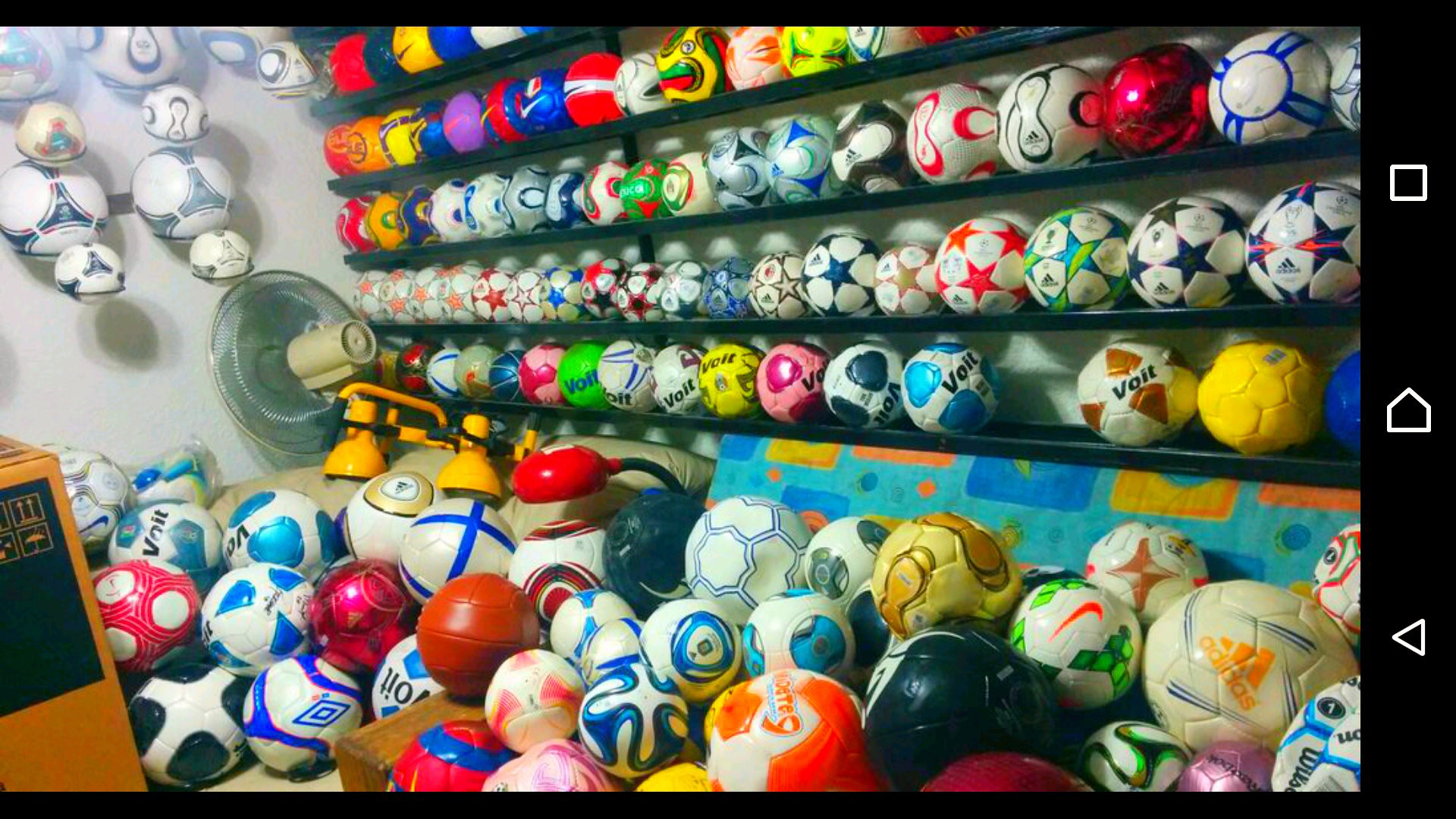The photograph depicts an indoor scene filled with a diverse collection of soccer balls. Central to the image is a black wall featuring multiple shelves—approximately five rows—each neatly lined with soccer balls of various sizes, designs, and colors, including red, blue, yellow, orange, pink, maroon, and gold. Notably, brands such as Nike, Adidas, and Voit are visible on many of the balls. On the lower part of the image, a pile of about 30 to 40 soccer balls lies on the ground, continuing the theme of abundant variety.

Adjacent to the black shelving, towards the left side, there's a white wall equipped with additional plastic shelves that also display more soccer balls. Above the scene, a fan is mounted and directed towards the back wall, possibly out of use as inferred from its position. In the lower left corner, a box marked with icons – including a black circle and an image resembling an umbrella – is partly visible.

Further details add to the richness of the scene: a colorful quilt with shades of blue, yellow, and orange is situated underneath the lower row of soccer balls. Black outlined circles, possibly a unique form of mounting or storage, hold some of the balls on the wall. Altogether, the scene creates a harmonious yet bustling display dedicated entirely to soccer balls.